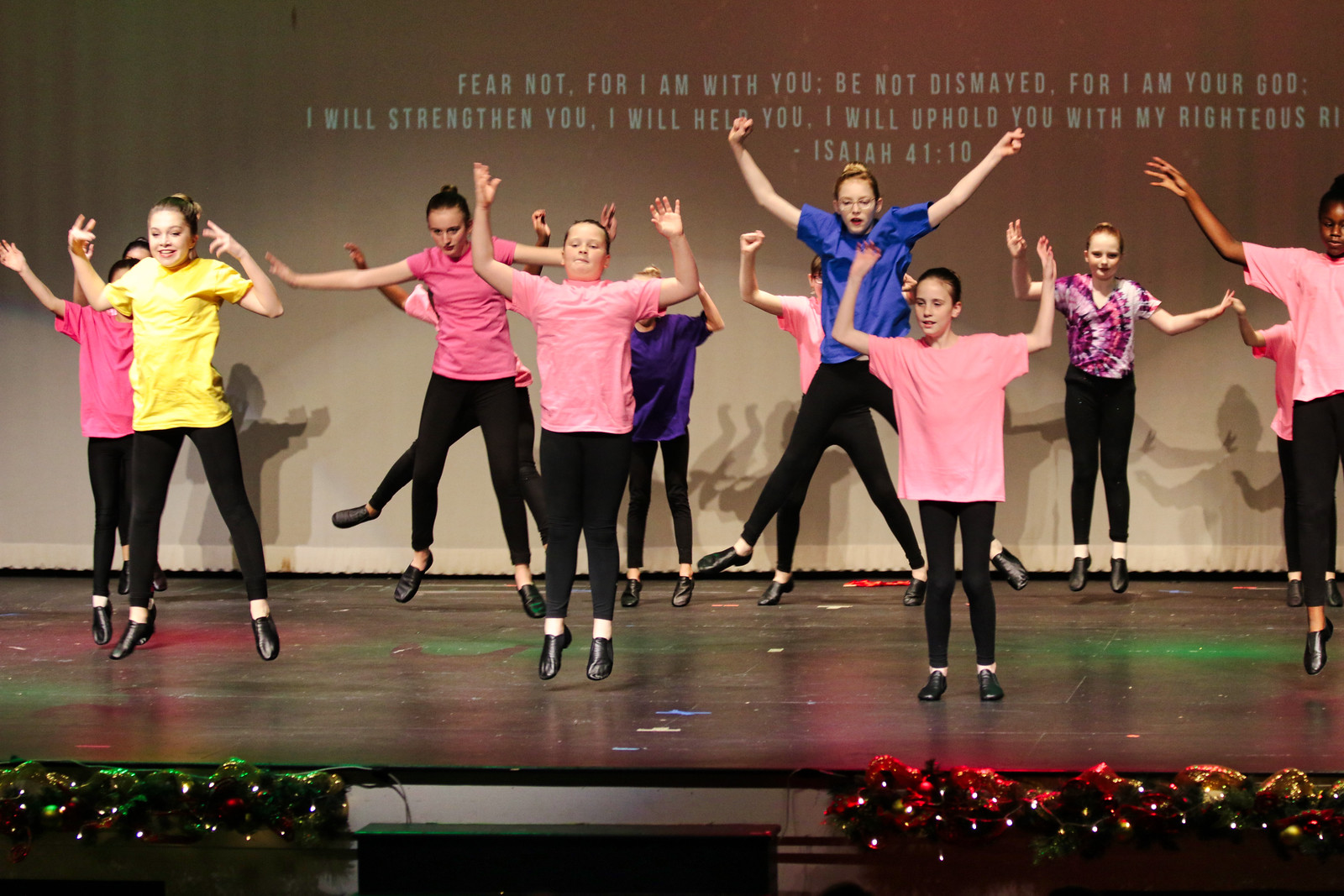This wide rectangular image depicts a group of young girls on a stage, dynamically captured in mid-performance, most of them leaping into the air with various poses. The stage has a sleek black surface that reflects the vibrant glow of green and red lights. At the front edge of the stage are darkly toned ornaments, likely red and white, accompanied by green Christmas wreaths on either side, adorned with colorful lights. In the center of the front row, a girl in a yellow shirt stands out among two others in pink shirts; notably, one pink-shirted girl at the right edge raises her arms instead of jumping. Additional rows of girls behind them similarly wear colorful shirts in hues of blue, purple, yellow, pink, and tie-dye, all paired with black leggings and ballet shoes. The backdrop features a beige curtain with an inspirational quote projected in white, capital letters: "FEAR NOT, FOR I AM WITH YOU. BE NOT DISMAYED, FOR I AM YOUR GOD. I WILL STRENGTHEN YOU. I WILL HELP YOU. I WILL UPHOLD YOU WITH MY RIGHTEOUS," which gets cut off, followed by "ISAIAH 41:10." The scene merges the festive decor and youthful energy into a cohesive moment of performance art.